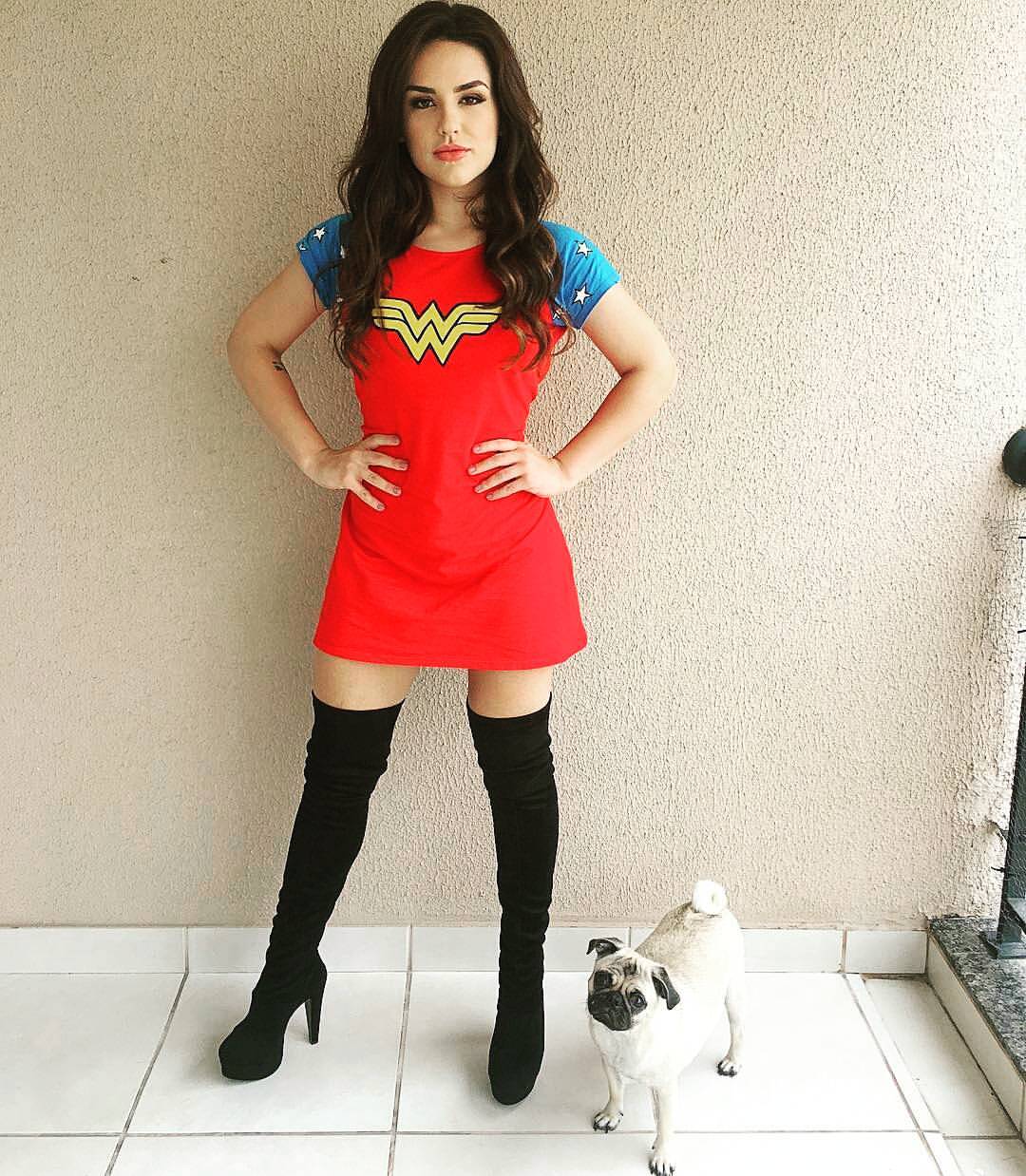In this photograph, a young woman exudes confidence as she stands in a powerful stance with her hands on her hips, wearing a striking Wonder Woman costume. The red mini-dress adorned with a gold Wonder Woman logo reaches midway down her thighs, complemented by blue sleeves decorated with white stars. Her long, wavy dark hair cascades just below her shoulders, contrasting with her fairly pale skin and dark brown eyes. Thigh-high black boots with high heels and platform soles complete her ensemble. To her right, a small pug with a black face, black eyes, and ears, but predominantly white fur, stands on an off-white tiled floor. The background features a cream-colored, textured wall, possibly hinting at an outdoor setting on a balcony, with natural light illuminating the scene from the right. The bottom part of a gate or a staircase railing is also visible in the frame.